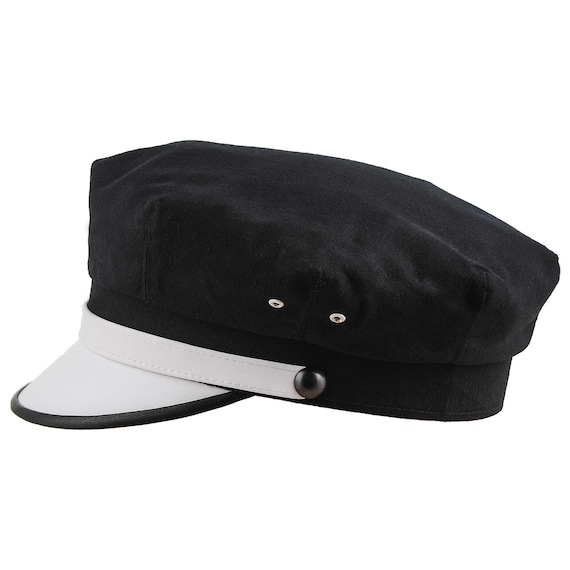The image displays a black hat, reminiscent of those worn by marching band members or boat captains, positioned sideways against a white background. The hat features a prominent white strip that runs across the front, fastened with a black button. The visor is white with a distinct black edge around it and extends only slightly. On each side of the hat, two small metallic rivets are visible, likely for ventilation. Simple in design yet formal in appearance, the hat also includes black banding, which wraps around the base to secure it on one's head. The overall presentation of the hat is zoomed in, providing a clear, detailed view of its features.